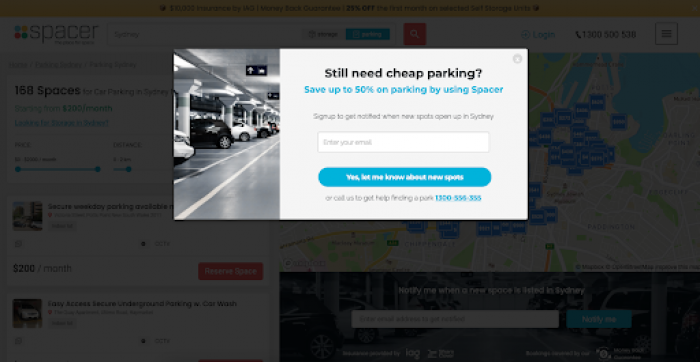This is a screenshot of a website displaying a prominent pop-up in the center. The pop-up is a white square with text and images. On the left side of the pop-up, there's an image of a parking garage featuring gray concrete columns and several cars, including white and black vehicles. The headline in black text reads, "Still need cheap parking?" followed by blue text stating, "Save up to 50% on parking by using Spacer." Below, black text invites users to "Sign up to get notified when spots open up in Sydney," with the last word being slightly difficult to read. There is an input box labeled "Enter your email" and a blue and white button that says, "Yes, let me know about new spaces." Gray and blue text, possibly including a phone number, is present at the bottom, alongside a gray 'X' to close the pop-up.

In the background, the website content is partially visible. On one side, "168 spaces" is written in black, accompanied by various filters. One spot is highlighted with a red box, indicating a price of $200 per month. 

At the top of the site, there's a gold banner with black text displaying the company name, Spacer. It includes a logo with colors purple, gold, salmon, and teal in overlapping circles. There is also a search bar, which is a white box with a blue box surrounding it and a red magnifying glass icon. Buttons labeled "Login" and a phone number, "1-300-500-538," are also visible. A map displaying tan and green land areas with numerous blue squares is shown. Further down, there is text reading "Notify me when a new space is available" alongside a white box and a blue button. No other significant details are visible in the image.